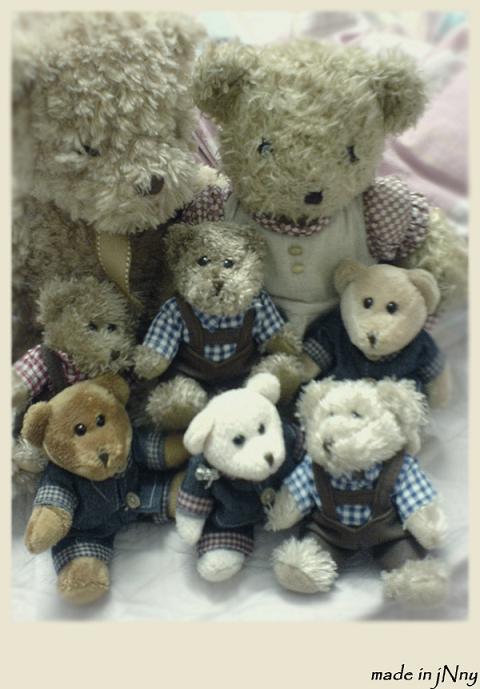This is a vintage-style Polaroid photograph featuring a teddy bear family arranged on a pink and white comforter adorned with designer patterns. The photograph has a thin white border, slightly thicker at the bottom edge. In the lower right corner, there is black text that reads "made in JNny," with 'J' and 'ny' in lowercase and the 'N' capitalized.

The central focus is a close-up of eight teddy bears, depicting a family scene. The two larger teddy bears in the back represent the parents; the left bear, presumably the father, wears a gold bow around its neck and has a gruff appearance. The right bear, presumably the mother, is dressed in a red checkered dress with short sleeves, a collar, and two buttons.

In front of the adult bears sit six smaller teddy bears, each with unique features and outfits. From left to right:
1. A light brown teddy bear with a gold bow around its neck.
2. A larger teddy bear dressed in checkered clothing, representing the mother, with a dress and vest.
3. A small teddy bear in a blue plaid shirt and overalls.
4. A white teddy bear in a blue denim bodysuit with red checkered sleeves and cuffs.
5. Another small bear with smooth, tan fur wearing a blue shirt with checkered sleeves.
6. A fuzzy white bear in a blue checkered shirt and dark overalls.

The teddy bears vary in fur texture, from shaggy to smooth, and in fur color, ranging from light brown to white. The intricate detail in their clothes, including checkered patterns and overalls, adds a charming, nostalgic quality to the scene.